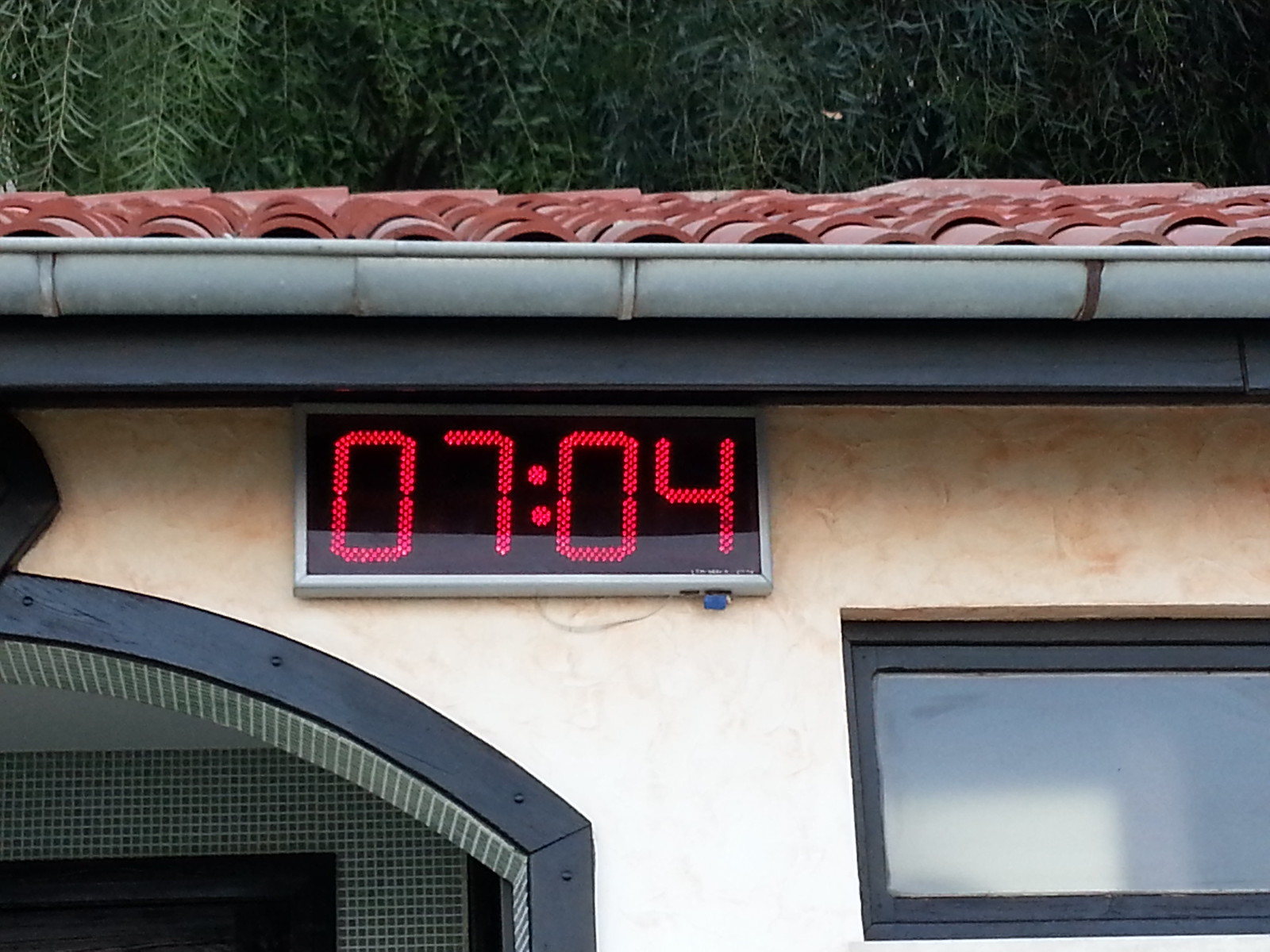This image depicts a charming cream-colored house with a distinctive terracotta slate roof. The roof tiles, resembling fragmented terracotta vases, add a vibrant red hue to the structure. A prominent digital clock displayed at the front shows the time as 7:04, without specifying whether it is a.m. or p.m.; however, the bright daylight suggests it is morning. Behind the roof, dense trees with weeping branches and fine, small leaves create a lush backdrop.

The stone exterior of the house, in a tan hue, includes a window with black trim and privacy glass, providing limited visibility through it. Below the clock, an electrical cord is visible, indicating its power source. The front door, set within an elegant archway, features a tiled entrance. The archway is brown with black paint, and the interior of the arch is lined with striking, elongated tiles, adding a unique architectural element to this picturesque residence.